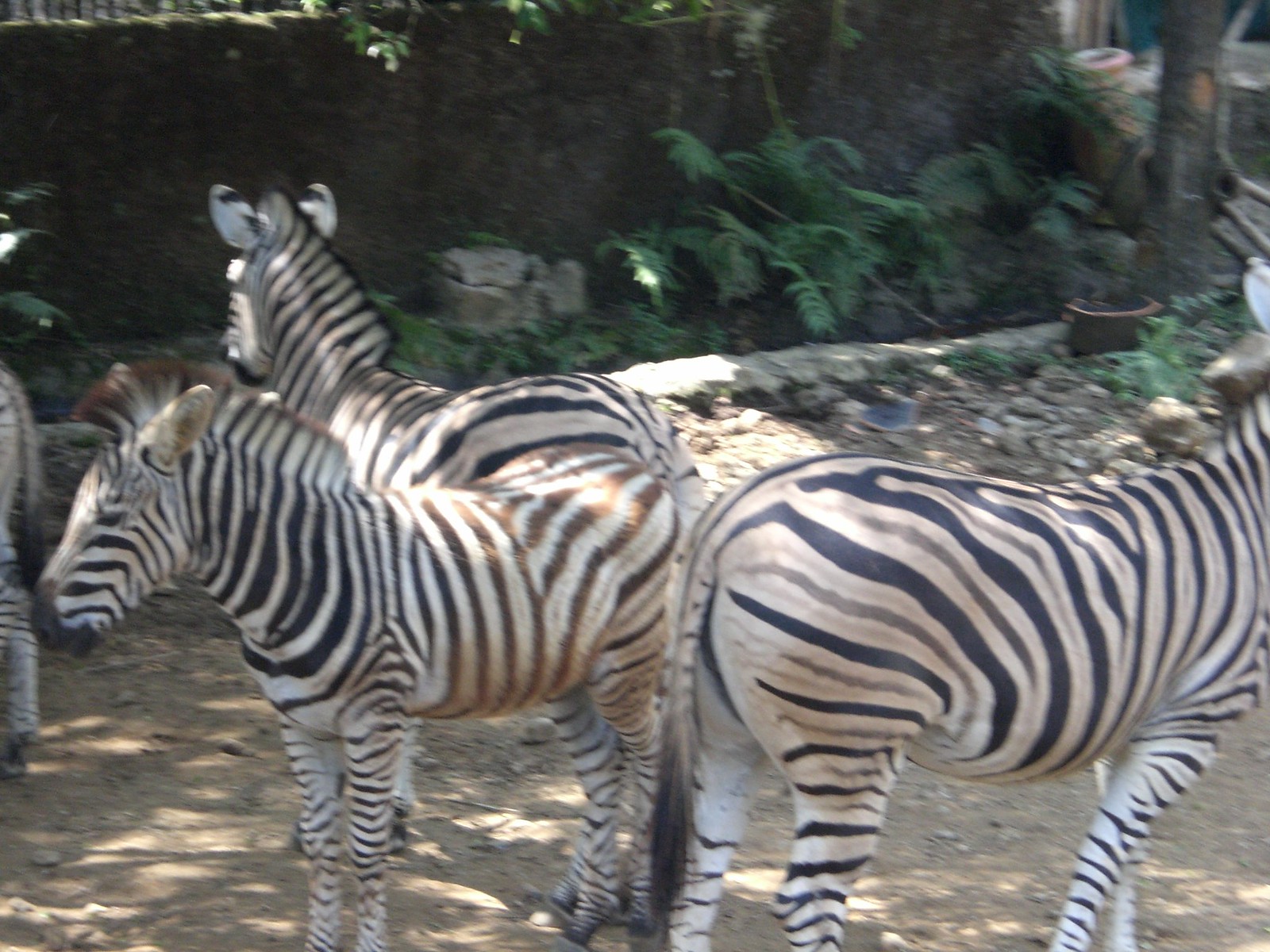This outdoor photograph, likely taken at a zoo, captures a slightly elevated view of three zebras standing on concrete ground, arranged in a spiral formation with their rumps facing inward. The image is slightly blurred and soft in focus, revealing two zebras in full with back stripes visible and the third zebra on the right partially cut off, missing its head in the frame. The environment behind them includes a mix of a dark brown dirt row with green plants growing out of it, and a stone wall or artificial construct that might be part of their enclosure. There's also a hint of a fourth zebra on the left, barely visible. The zebras show signs of dirt on their bodies, indicating they have been rubbing against the ground, and the overall lighting is dim due to the photograph's quality. Additionally, flower pots are visible in the background near a drop-off filled with greenery.